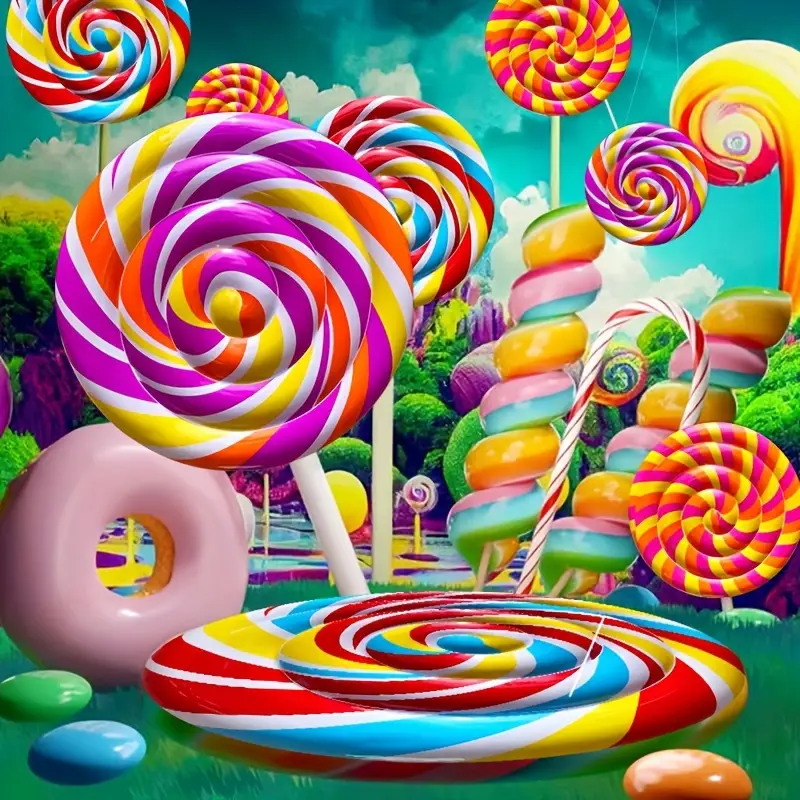The image is an overwhelmingly colorful depiction of a whimsical Candyland. Dominating the scene are gigantic, swirling lollipops in an array of vibrant colors, including combinations of white, yellow, purple, orange, red, blue, and green. Some of these lollipops are planted into a vivid green lawn, standing taller than the surrounding trees, while others seem to soar into a bright blue sky adorned with fluffy white clouds. Scattered throughout the landscape are various candy-themed elements: a large pink donut on the left side, multi-colored pieces of candy resembling M&Ms, and vertical, swirly candy confections in hues of pink, blue, green, and yellow that stretch towards the heavens. Additionally, colorful eggs—orange, blue, and green—dot the ground, enhancing the fantastical, mouth-watering nature of this candy paradise.